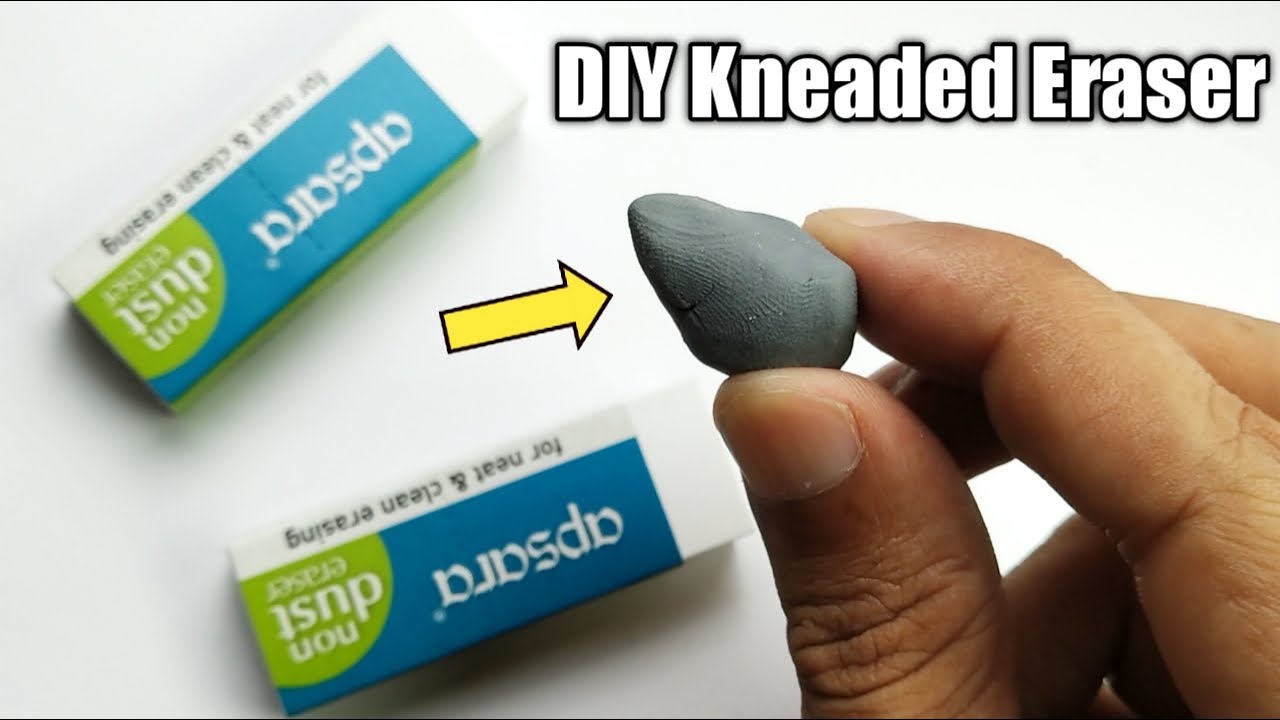This image, possibly taken from a YouTube thumbnail, presents a step-by-step guide to creating a DIY kneaded eraser. The background is white and predominantly horizontal in format. The upper right-hand corner has text in a bold, white impact font with a black outline and shadow reading "DIY Kneaded Eraser." Central to the image is a person's hand emerging from the bottom right corner, holding a gray substance that appears to be clay or Play-Doh, molded into a teardrop shape with visible thumbprints. This gray object is highlighted by a yellow arrow with a black outline pointing towards it, indicating its significance. 

In the same scene, two upside-down packaging boxes are situated on the left, described as white with blue and green elements and labeled with "for neat and clean erasing," though the brand, presumably Apsura, is challenging to decipher. The overall composition and text appear to inform viewers on how to transform regular non-dust erasers into a customizable kneaded eraser.